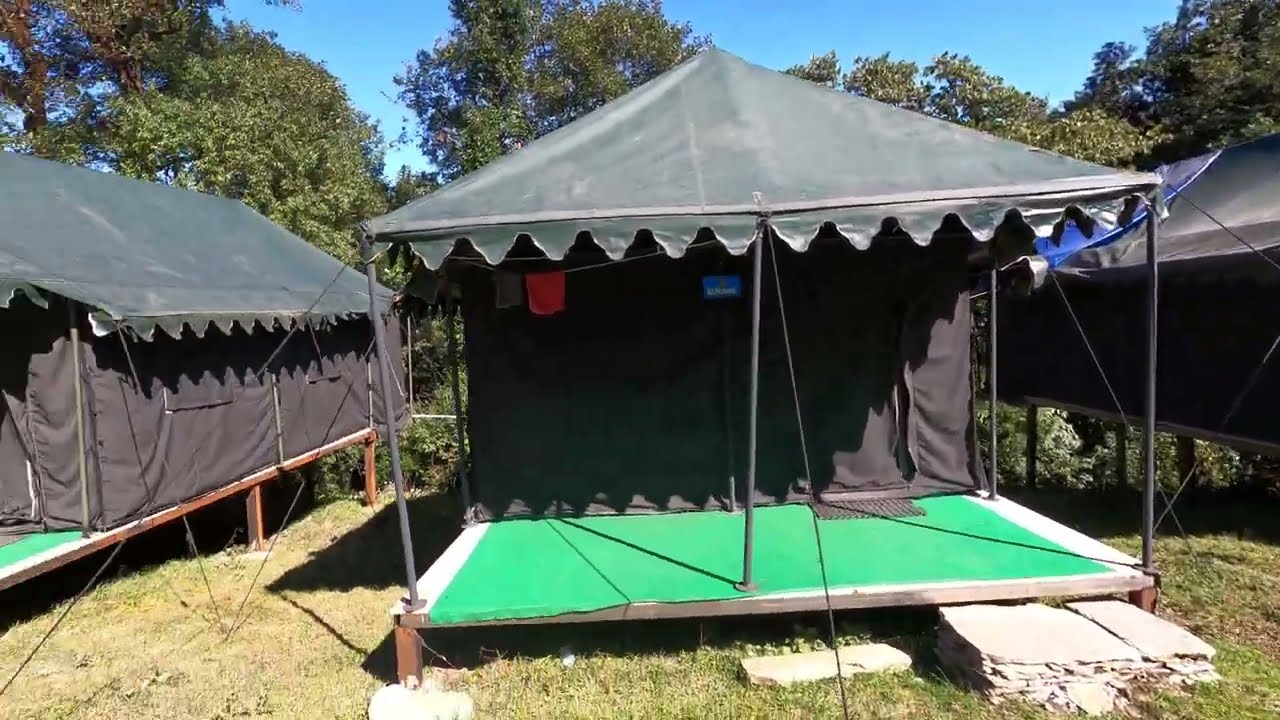This photograph captures a serene campsite featuring three prominent black canvas tents, each set up on elevated wooden platforms. The central tent dominates the frame, with identical tents flanking it on both the left and right sides. Each tent includes a small porch or patio area, furnished with a green mat, extending a couple of feet from the edge of the platform. Tiny poles and flat rocks provide support and structure for these semi-permanent fixtures. Festive red flags or banners dangle beneath the makeshift porches, adding a touch of color to the campsite. In the backdrop, a clear, cloudless blue sky arches over several large trees, casting intermittent shade on the patchy grass and rocky ground below. The sunlight bathes the entire scene, highlighting the tranquility and organized simplicity of this secluded outdoor retreat.